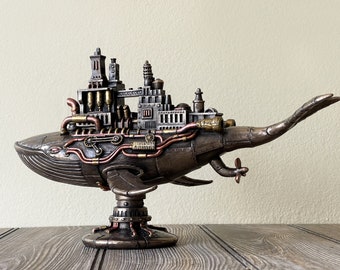This image depicts a steampunk-inspired sculpture of a whale, featuring a blend of mechanical and marine elements. The whale appears to be constructed from materials that give it a copper and bronze hue, with intricate details such as gears, pipes, and propellers integrated into its design. On its back rests a large cityscape, complete with buildings, giving the impression of an entire city being transported. The sculpture is mounted on a circular stand with a flat base, allowing it to stand upright on a medium brown wooden table. Threads of copper wire intertwine throughout the whale, adding to its mechanical aesthetic. The underbelly of the whale showcases a metallic gray-silver tone, complemented by twin tails at the back. The background is a plain white wall, providing a neutral backdrop that highlights the intricate details of the sculpture.